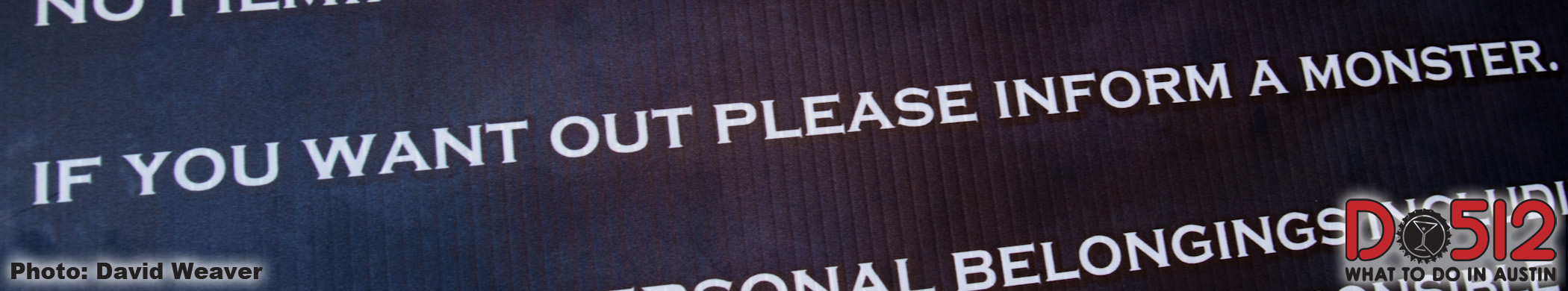The image displays a rectangular sign with a black background featuring bold white text. The most prominent line, centrally placed, reads: "If you want out, please inform a monster." Above this line, partially obscured, is the word beginning with "no." The bottom left corner identifies the photographer with, "Photos: David Weaver," using black text with a white glow. In the bottom right, there’s a logo with a capital letter "D" adjacent to a black circle containing a martini glass. Next to this, red text spells "512." Below the logo, black text with a white halo states, "what to do in Austin." Hints of color variations and potential background design elements such as dark blue transitioning to brown and red are suggested but not clearly defined.